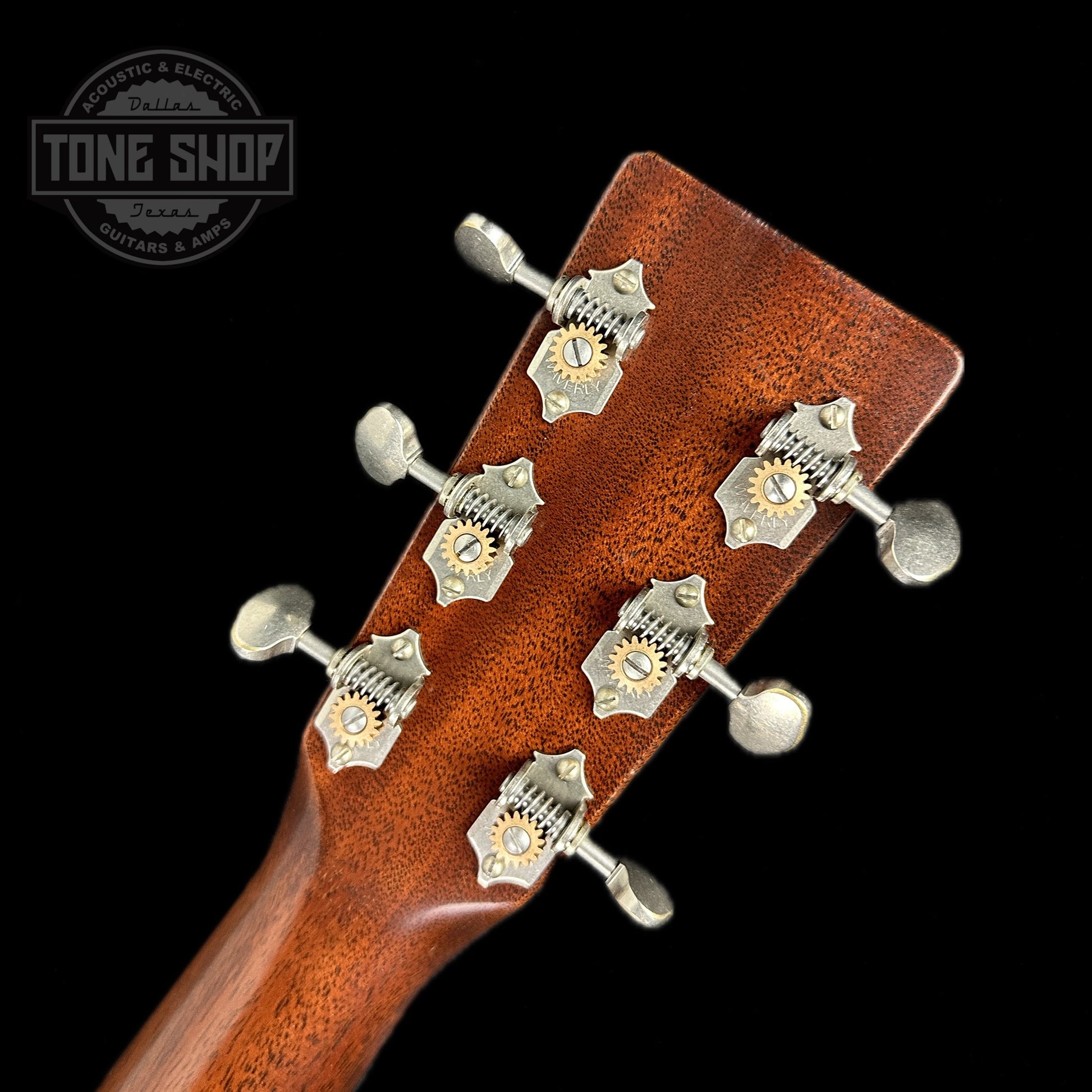This image features a detailed close-up of the head and neck of a highly polished, reddish-orange wooden guitar, set against a stark black background. Prominently, it showcases six silver tuning mechanisms with gold gear-like pieces around screws, which interlock with the strings to allow for precise tuning. In the top left corner, the Tone Shop logo is visible—a gray circle intersected by a rectangular box, with the text "Tone Shop" inside it. Below, the logo further reads "acoustic and electric guitars and amps," indicating the shop's origins from Dallas, Texas.